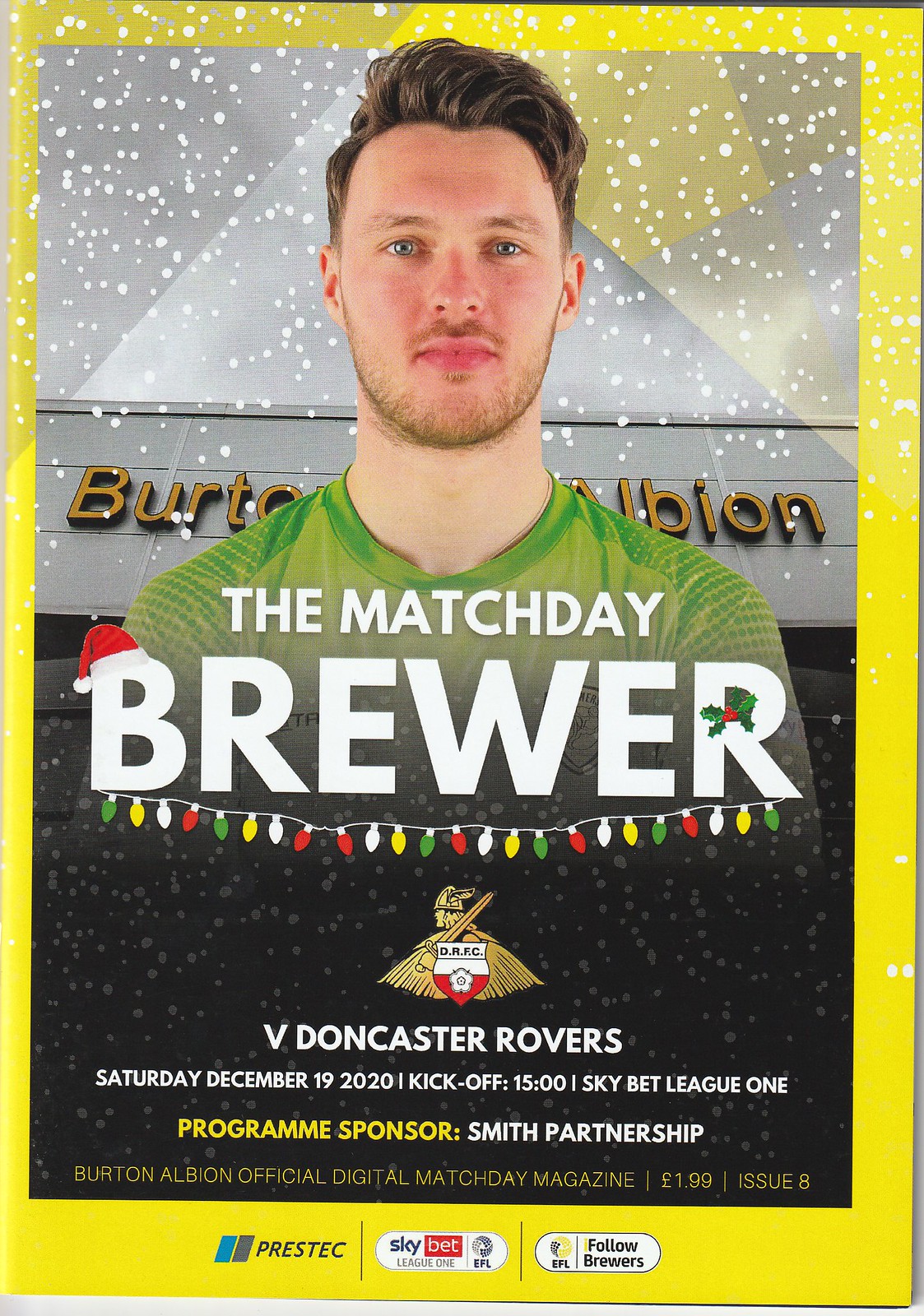The cover of the Burton Albion Official Digital Match Day Magazine is adorned with festive elements and vibrant details. At the top, "The Match Day Brewer" is prominently displayed in white text over a green jersey, worn by an unidentified soccer player with brown hair, blue eyes, and a stoic expression. Adding a touch of holiday cheer, the 'B' in "Brewer" wears a Santa cap, and the 'R' is decorated with mistletoe, while multicolored Christmas lights (white, yellow, green, and red) hang between them. Below the title text is an emblem, followed by details of the event: "V. Doncaster Rovers, Saturday, December 19th, 2020, Kickoff 1500, Sky Bet League One." The program sponsor, Smith Partnership, is acknowledged in yellow text, and at the bottom, various logos, including Prestec and EFL, are visible, along with the price of £1.99 and the issue number eight. The magazine features a yellow border, with the central area depicting geometric silver shapes and a black background, partially obscured by the soccer player, evoking a wintry scene with white dots resembling falling snow.